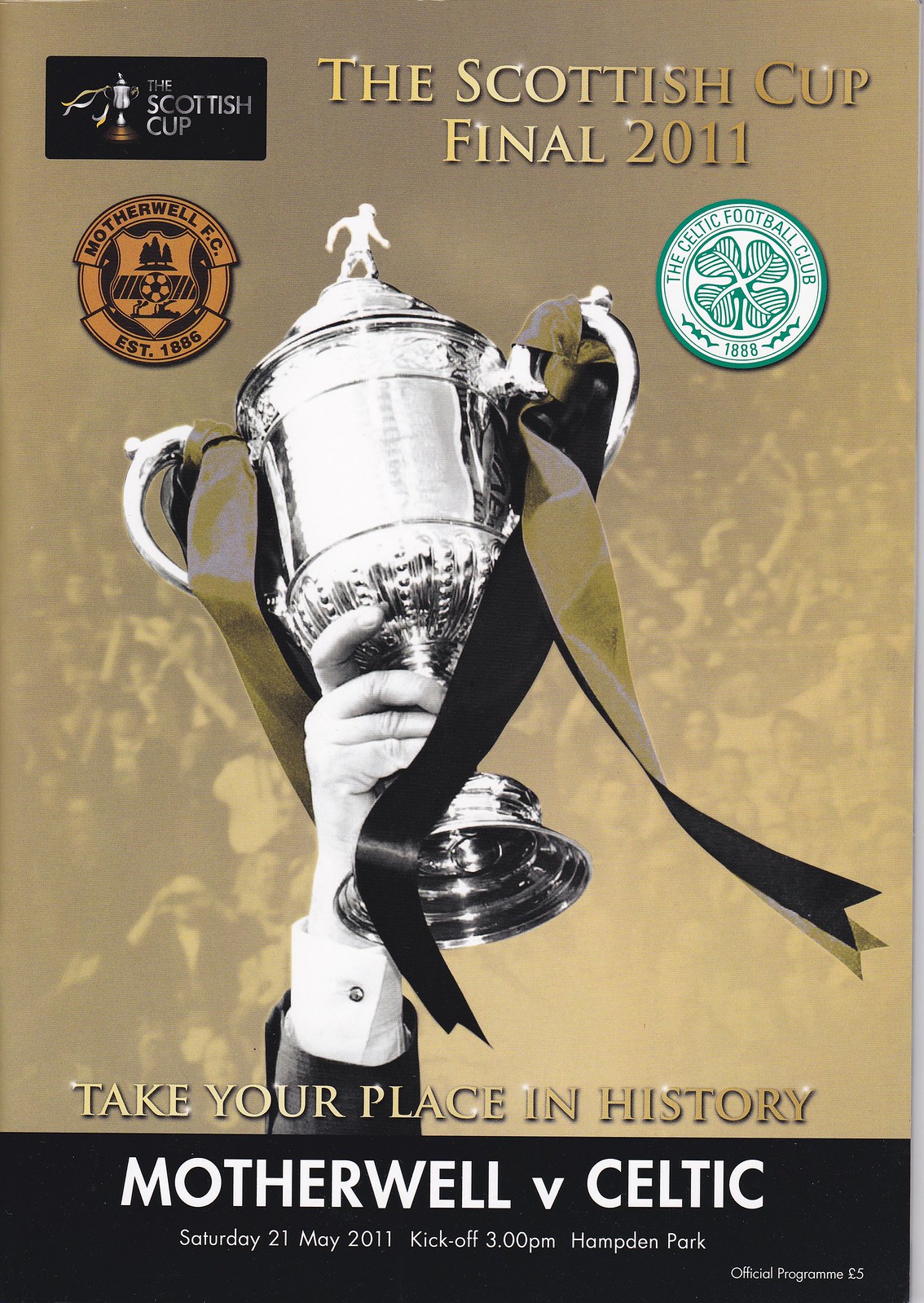The cover of the soccer program for the Scottish Cup Final 2011 features a golden brown and black theme depicting a blurred crowd in the background. Dominating the center is a black and white photograph of a hand triumphantly holding up the silver Scottish Cup adorned with gold and black ribbons. In the top left corner within a black rectangle, the Scottish Cup logo is displayed. Alongside it in bold gold lettering is "The Scottish Cup Final 2011." Flanking this are badges; on the left is the emblem of Motherwell FC with its founding year, 1886, and on the right is the green and white circular badge of Celtic Football Club featuring a clover and the year 1888. Beneath the central image, the gold text reads "Take Your Place in History." A black band at the bottom of the cover with white text announces "Motherwell vs. Celtic, Saturday 21st May 2011, Kickoff 3 p.m., Hampden Park." In small print at the very bottom, it states "Official Program" and "£5."